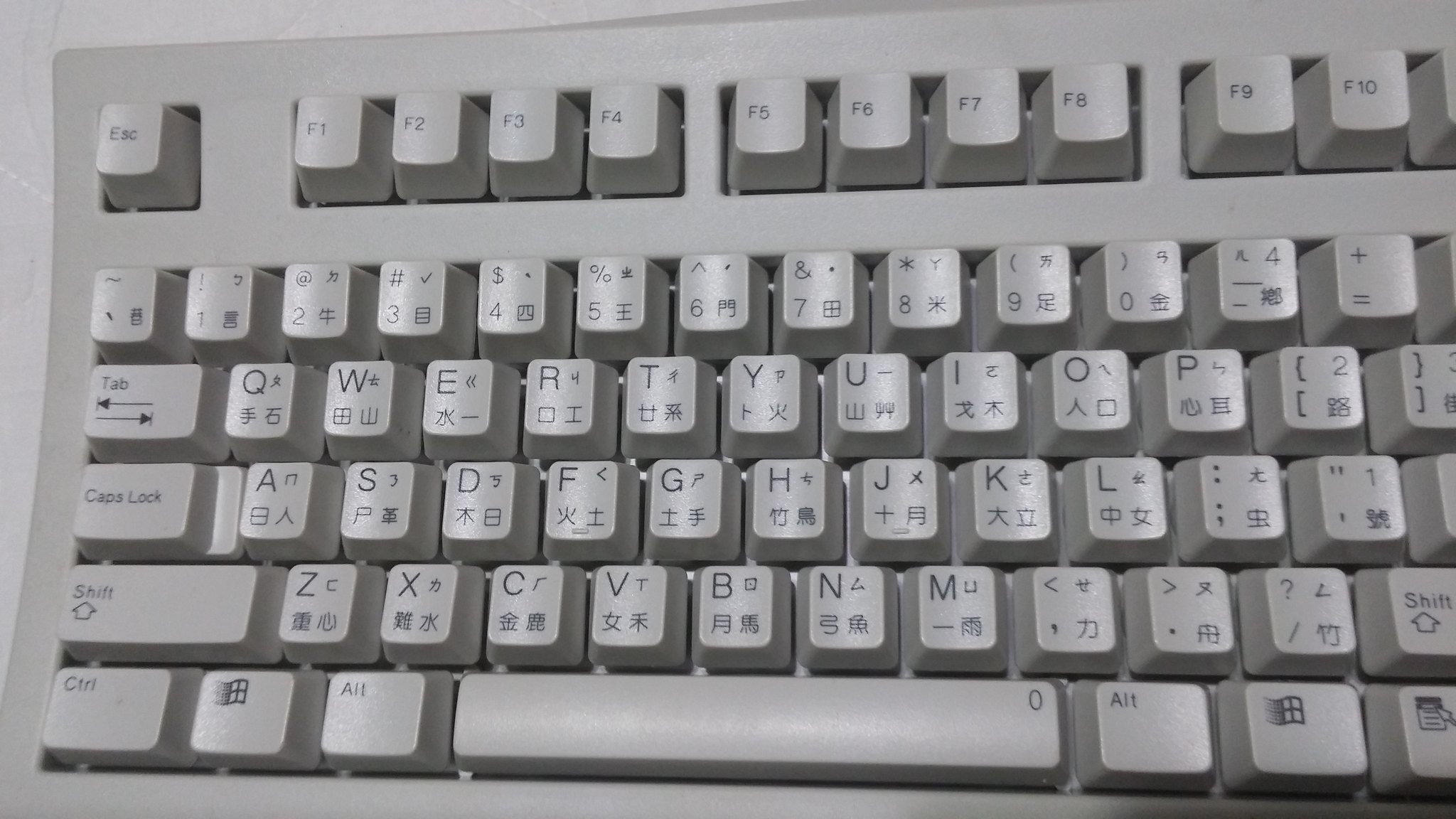This realistic photograph, oriented horizontally, features a vintage, off-white to gray computer keyboard, presumably from the early 2000s. The main focus is on the left 80% of the keyboard, extending from the Escape key and F1 through F10 keys on the top row down to the QWERTY layout with standard English keys complemented by Asian characters, likely Japanese, evidenced by the presence of hiragana, katakana, and possibly kanji symbols. The keyboard combines English letters and Asian characters on each key, including punctuation marks and numbers, and features fat, distinct keys like Tab, Caps Lock, Shift, and Control, as well as a spacebar marked with a zero. A Windows key indicates it’s designed for a Windows operating system. The background shows a light gray tabletop visible on the left and top edges, enhancing the keyboard's aged appearance as if sun-exposed over time.